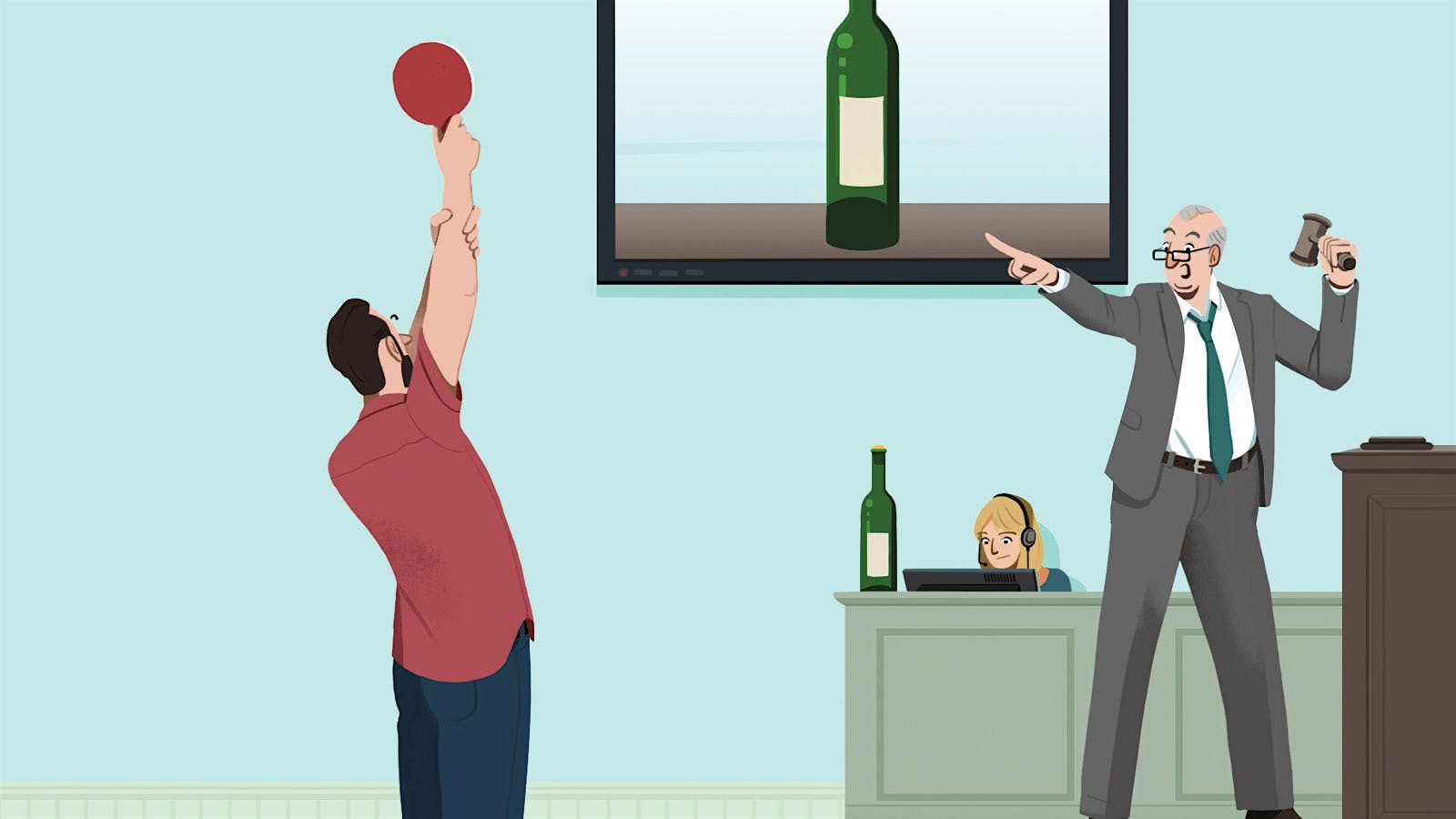In this animated, cartoon-stylized illustration set against a plain light blue wall, three distinct characters are depicted in an office-like setting. In the background, a blonde woman wearing headphones sits at a desk, intently looking at a computer screen; an apparent receptionist or possibly a court reporter. A green bottle, resembling a wine or cider bottle, is placed on her desk, and above her, a large photograph of the same bottle hangs on the wall.

In the foreground, a tall, slightly balding man with glasses and a small beard stands, dressed in a gray business suit with a greenish-blue tie. Holding a gavel and standing near the edge of what resembles a judge's desk with a gavel pad visible, he points assertively at another man. This second man is positioned to the left, wearing a red shirt and blue jeans, with brown hair and a beard. He raises a red table tennis paddle in his right hand while gripping his forearm with his left, as if making a bid. The overall scene appears to be a lively auction, with the gavel-bearing man potentially serving as the auctioneer of the featured green bottle.